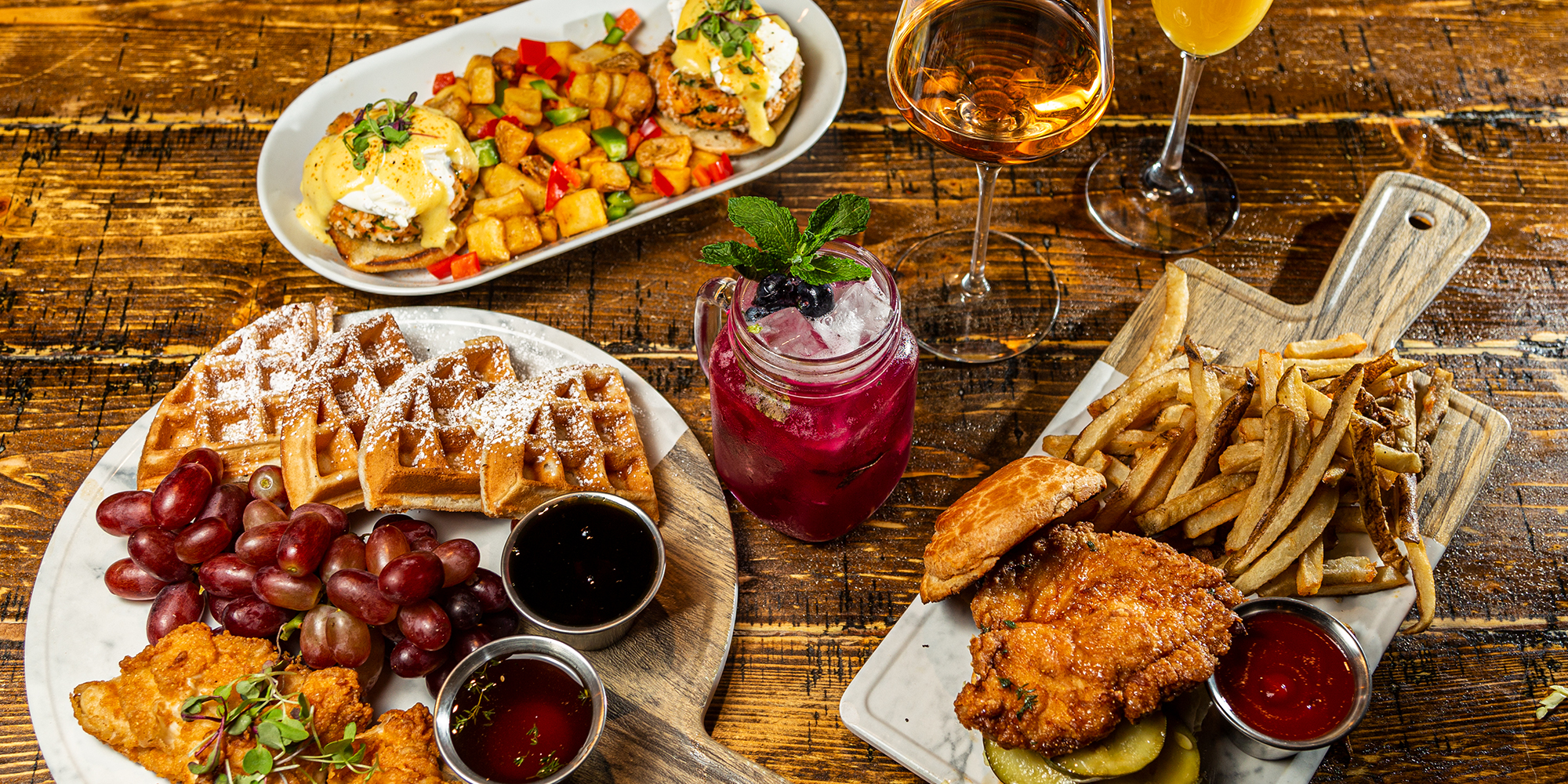This image captures a rustic wooden table laden with an assortment of food and drinks. Centrally positioned is a mason jar filled with a reddish liquid, ice cubes, and a sprig of mint, possibly a fruit-infused drink. Flanking the mason jar are two glasses: one is a wide, clear wine glass containing an amber liquid, likely apple juice, and the other is a thin wine glass filled with an orange liquid, possibly mimosa or orange juice.

To the upper left, there is an oval white plate featuring an array of diced potatoes and peppers in the center, flanked by two sandwiches with eggs and light brown meat topped with green peppers. Below it, to the left corner, a circular wooden tray with a handle holds four waffle quarters dusted with powdered sugar, a cluster of purple grapes on the stem, and two silver canisters likely containing syrup and perhaps another sauce for the accompanying garnish-topped fried chicken.

On the right, a rectangular wooden serving board with a handle displays a large chicken sandwich with pickles beneath the chicken, the top bun off to the side. Above the sandwich, a pile of hand-cut fries is served next to a small metal tin of ketchup, creating a hearty and diverse spread representative of a satisfying feast.